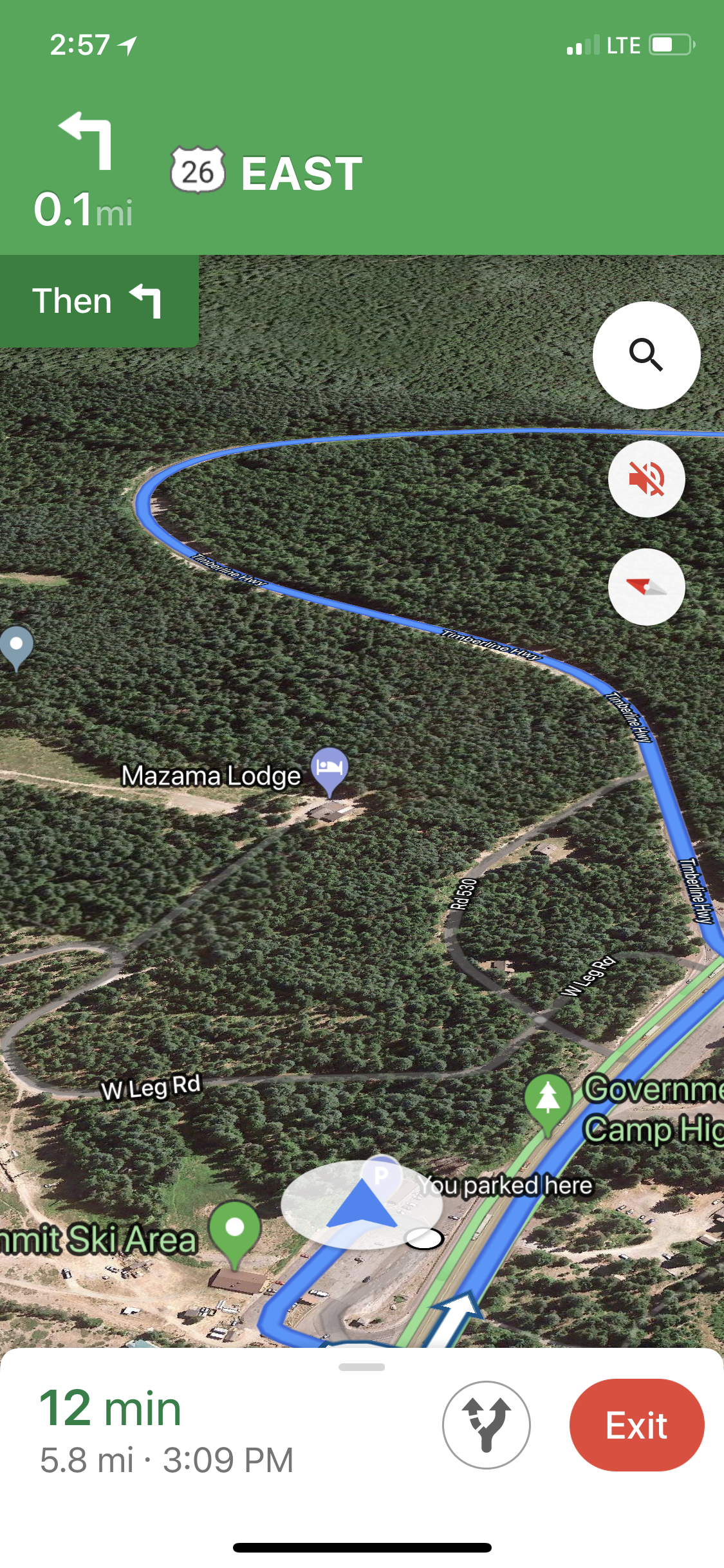The image is a detailed screenshot from a smartphone showing directions on Google Maps with an aerial view. The background prominently displays trees, roads, and landmarks, such as Summit Ski Area and a government campground marked with teardrop-shaped icons. A green highway sign at the top indicates the user needs to take Highway 26 East, with a left turn required in 0.1 miles. Overlaying the aerial photo are blue lines marking the intended route, with names of roads and points of interest clearly labeled, including Westleg Road and Mazama Lodge, symbolized by a bed icon. The lower portion of the image displays navigation details, including the estimated travel time of 12 minutes over 5.8 miles, with an arrival time of 3:09 PM. Additional icons show signal strength, LTE connection, battery status, sound settings, and search functions. A red exit button is visible at the bottom right, allowing the user to exit the navigation program.